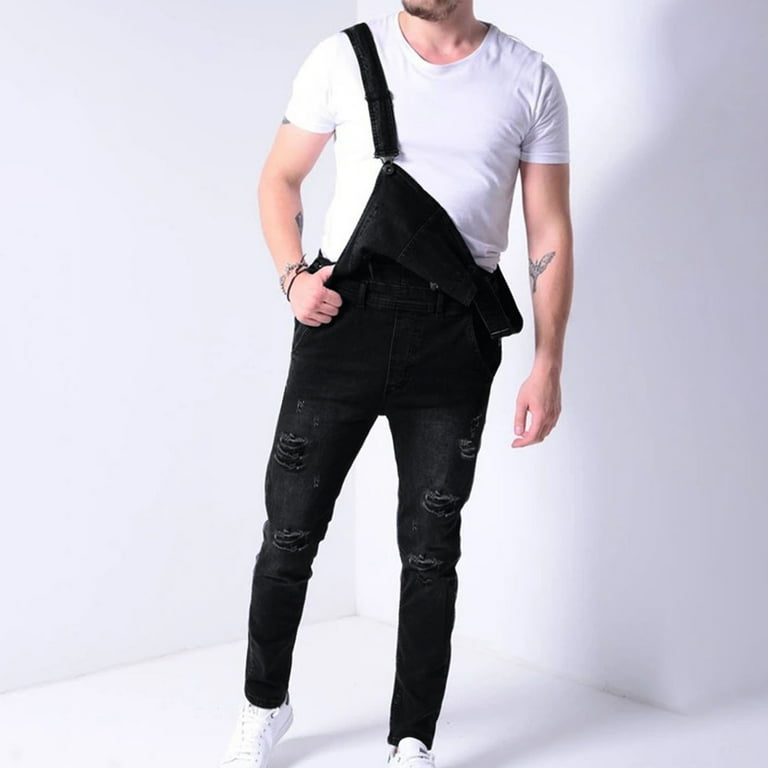This color photograph captures a muscular man from the chin down, modeling a black apron slung over one shoulder. The second strap of the apron hangs loosely by his left side, with his thumb cupped into the apron and held by his right hand, while his left hand hangs loosely by his side. He wears a white short-sleeved t-shirt, black torn jeans with tears on the knees and upper thighs, and white tennis shoes. His forearm features tattoos, including a prominent butterfly on his left arm. The man stands in a white room that casts his shadow to the right, emphasizing the stark contrast between his attire and the background.